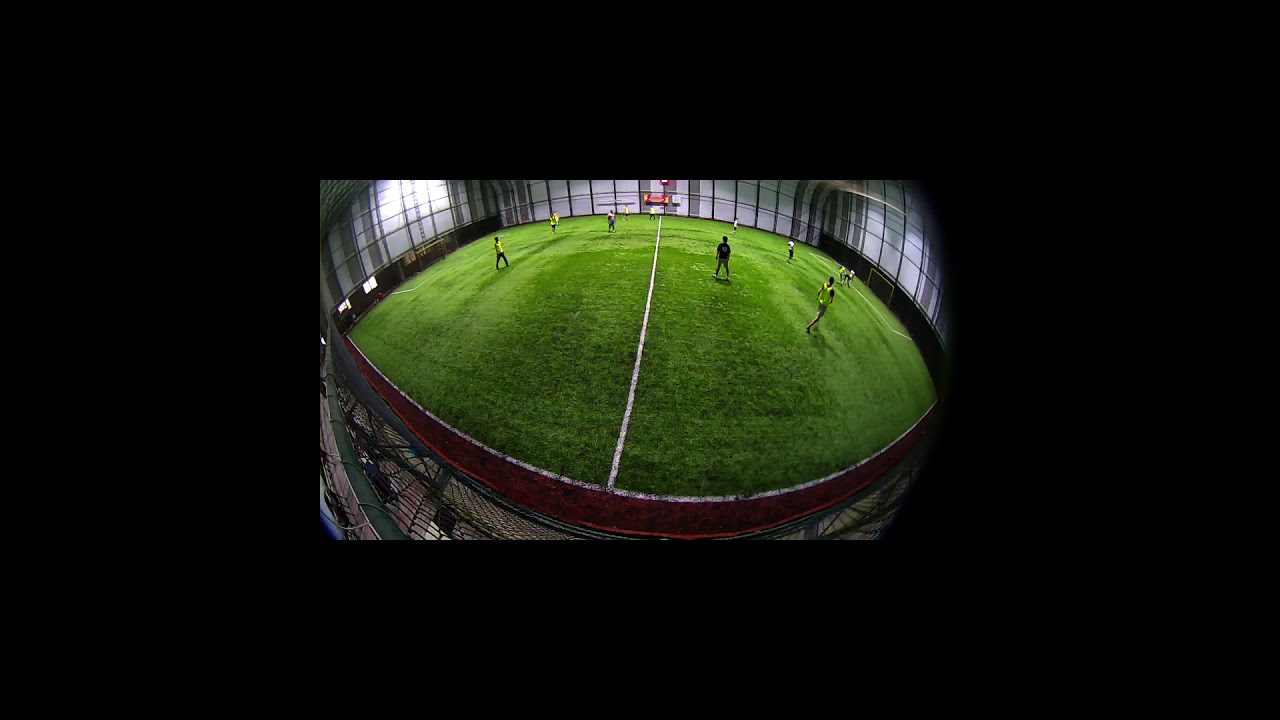This is a photograph showcasing an indoor soccer match, captured from a high vantage point, likely resembling a security camera or a panoramic view, which gives it a slightly distorted, rounded appearance around the edges. The photograph is positioned centrally within a rectangular black mat that borders the image. 

The field's green surface, possibly vibrant turf, is enclosed by a fence featuring a red top and black frame. A prominent white line runs down the middle of the field, with additional white lines marking the boundaries. The arena itself has white and gray walls, and visible goalposts on either side of the field are yellow.

There are various players on the field, notable by their yellow and white uniforms, engaging in mid-play. Despite the presence of goalposts, no one is actively guarding them. The background includes signs on the far wall, one of which is red with some yellow accents, and two white signs, though the specifics are indistinguishable due to the distance. Overall, the absence of spectators suggests this could be a practice session rather than an official match.